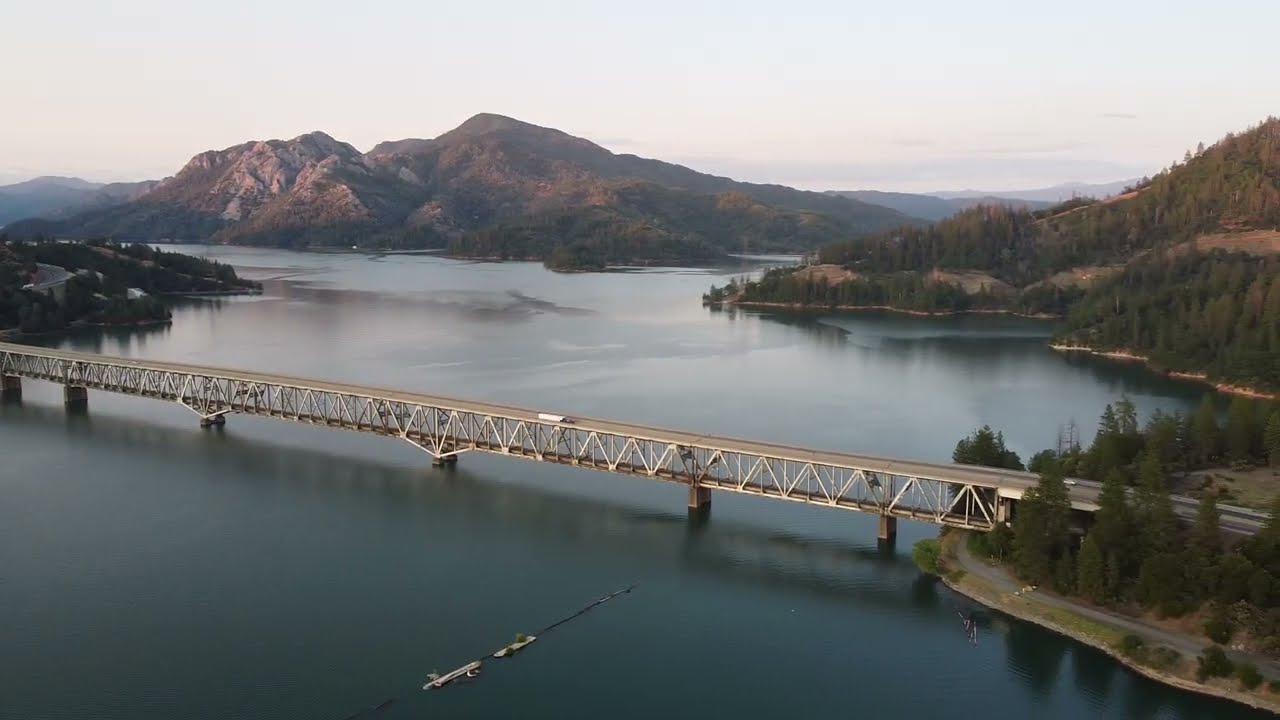This aerial photograph showcases a serene, expansive lake with glassy, dark waters, nestled amidst rugged, jagged mountains clad in rich greenery and rocky outcrops. A striking white, two-level bridge, supported by large concrete structures, elegantly stretches across the lake, connecting the mountainous shores. The bridge, made out of metal, carries both vehicles, including visible trucks, buses, and cars on the top level, while potentially accommodating trains on the lower level. In the foreground, the calm lake features some small watercrafts near the bridge. Surrounding the lake, a perimeter road winds through dense forests of redwood or pine trees, extending from the mountain slopes down to the water's edge, adding to the picturesque, almost unspoiled landscape.